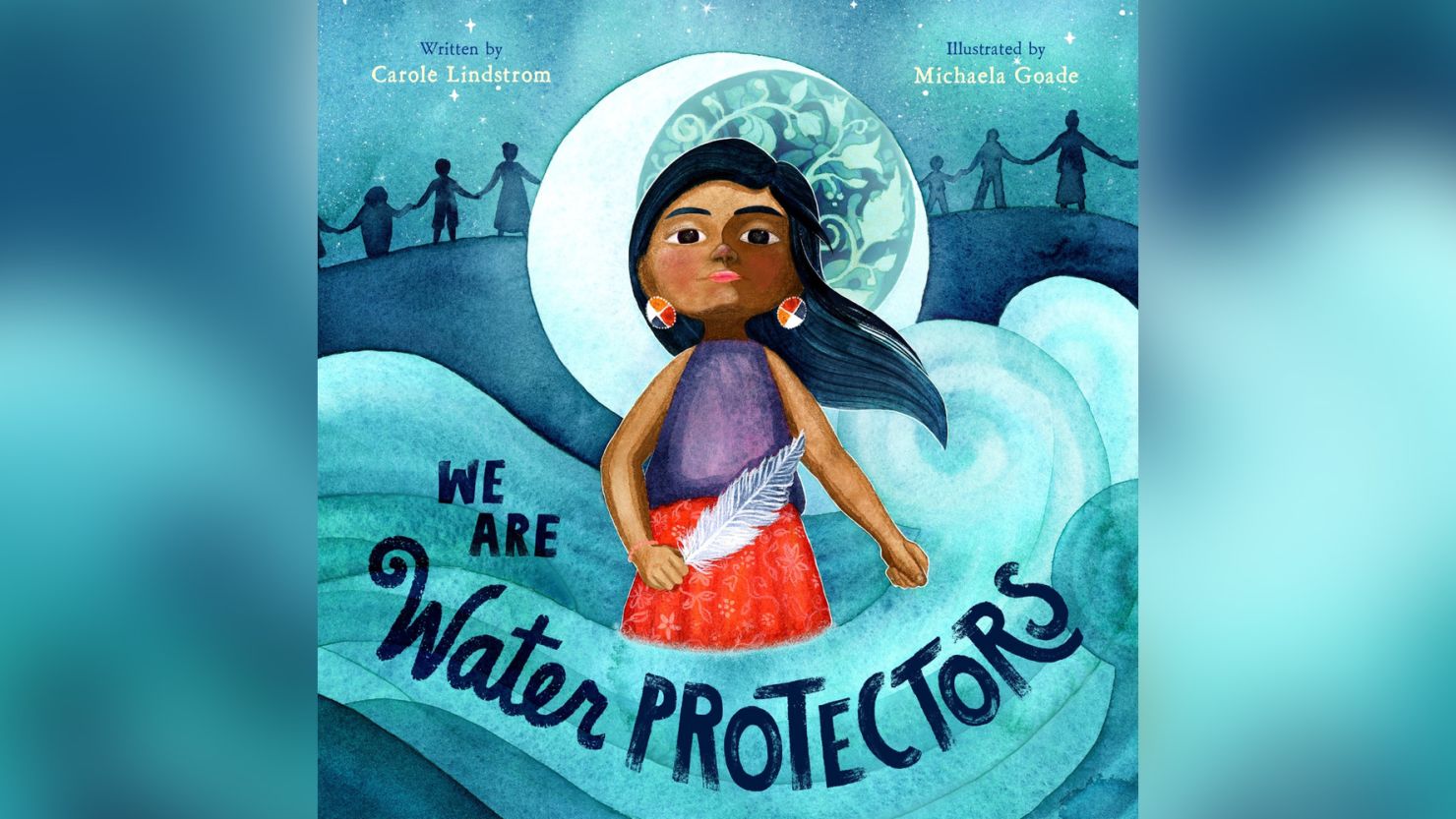The rectangular horizontal image, reminiscent of a book or comic cover, features a detailed illustration centered amid blue hues that range from light to dark. The left and right edges of the image blend into a blurry, ethereal background of swirling, light blue wind patterns. Central to the composition is a striking drawing of a Polynesian woman, who stands poised with long, flowing dark hair and elaborate, multi-colored triangular earrings. She wears a purple sleeveless top paired with a red skirt that matches her orange lipstick. The woman holds a white feather in her left hand, symbolizing purity and peace.

Encircling her legs is a billowing, cloud-like formation with the text "We Are Water Protectors" prominently displayed below her. Above her head floats a celestial backdrop featuring a crescent moon integrated with intricate designs of plants and flowers. The names of the creators, Carol Lindstrom and Michaela Gold, are subtly included, suggesting the image serves as a cover illustration for their collaborative work. In the background, there's also a holding of hands that symbolizes unity and solidarity.